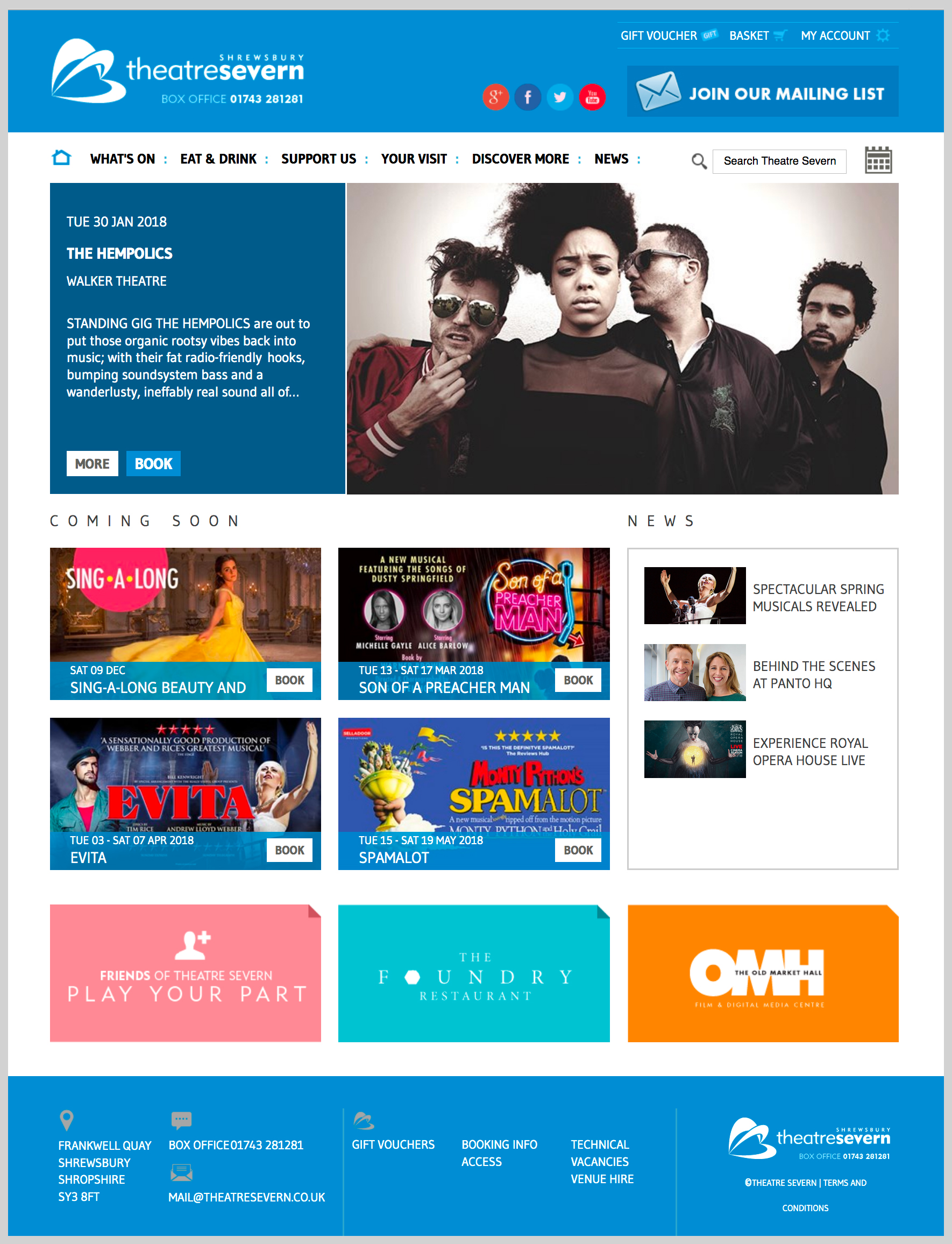This image is a full-color screenshot of Theodor Severn's website. The top section features a blue background with an icon resembling a heart-shaped page being turned, symbolizing perhaps a book or a newsletter. Prominently displayed are social media icons for Facebook and Twitter. There is a call-to-action area with a blue button labeled "Join Our Mail List," accompanied by an envelope icon.

The website's main navigation includes headings in bold black font, such as "What's On," "Eat and Drink," "Support Us," "Your Visit," "Discover More," "News," and a search function. Several sections with visual content are displayed below. The topmost group photo showcases four individuals - one woman and three men. Directly below this image, a heading reads "Coming Soon," followed by "News."

A notable feature in the "News" section is an image of a sing-along event, highlighting a lady wearing a vibrant yellow flowing dress. Additional content includes details about upcoming shows like "Evita" and "Spamalot," alongside other event information.

The bottom of the webpage is bordered with a blue strip containing white text. Overall, the website serves as a dynamic platform to promote various events and activities offered by Theodor Severn.